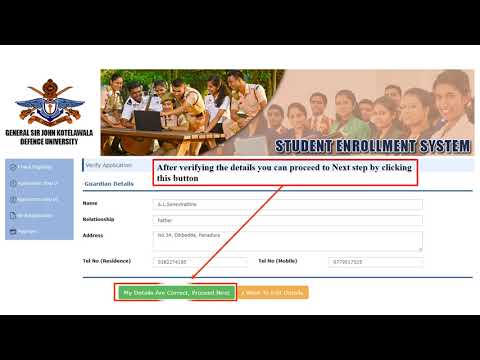The image has a white background with two thick black bars at the top and bottom. On the left side of the image, there's an icon followed by the text, "General Sir John Kotelawala Defence University." To the right of this, there are two side-by-side pictures.

In the picture on the left, a group of six people stands around one person seated at a picnic table bench. They are all focused on a computer. This scene suggests a collaborative setting, possibly involving a demonstration or training.

The picture on the right shows seven or eight people facing the camera, hinting at an organized group. The location appears to be somewhere in India.

At the bottom of the right picture, in all caps text, it states, "STUDENT ENROLLMENT SYSTEM." Below this caption, there's a red-outlined box containing text that directs, "After verifying the details, you can proceed to the next step by clicking this button." This message points to a blurry green button, which is unreadable, next to an equally blurry orange button that appears to have the label "Guardian Details."

Further down, there are labeled fields for "Name," "Relationship," "Address," "Telephone Number (Residence)," "Telephone Number (Mobile)," and spaces for writing information, though the details are indistinguishable due to the blurriness.

On the left side, a blue box with five lines of text is completely unreadable, adding to the overall unclear details within the image.